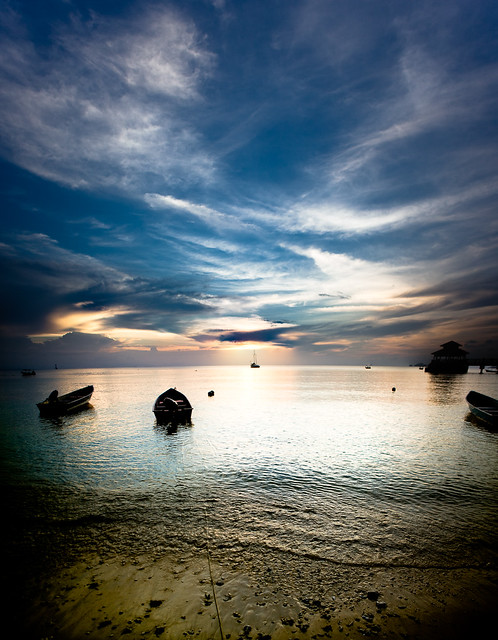This vertically oriented photograph captures a serene, early evening scene outdoors by a tranquil body of water, possibly an ocean or a lake. At the bottom of the image, the shore features packed sand interspersed with rocks that display a yellowish-tan hue, possibly due to algae. Gentle, small ripples of water move toward the shore, contributing to the calm atmosphere.

In the midsection of the photo, several small boats, likely canoes, are scattered across the water. One is positioned on the left side, another near the middle, and a part of one is visible on the right, with an additional boat seen far off in the distance. To the right, part of a building is noticeable, adding a subtle human element to the natural scene.

The upper portion of the image showcases a striking sky, transitioning from a dark blue at the top to an orange and yellow gradient near the horizon, suggesting the sun is either setting or rising behind a cluster of feathery white clouds. This vivid contrast is reflected subtly on the water’s surface, enhancing the image's overall beauty and depth. The horizon line is horizontally centered, visually balancing the composition between the sky, water, and shoreline.